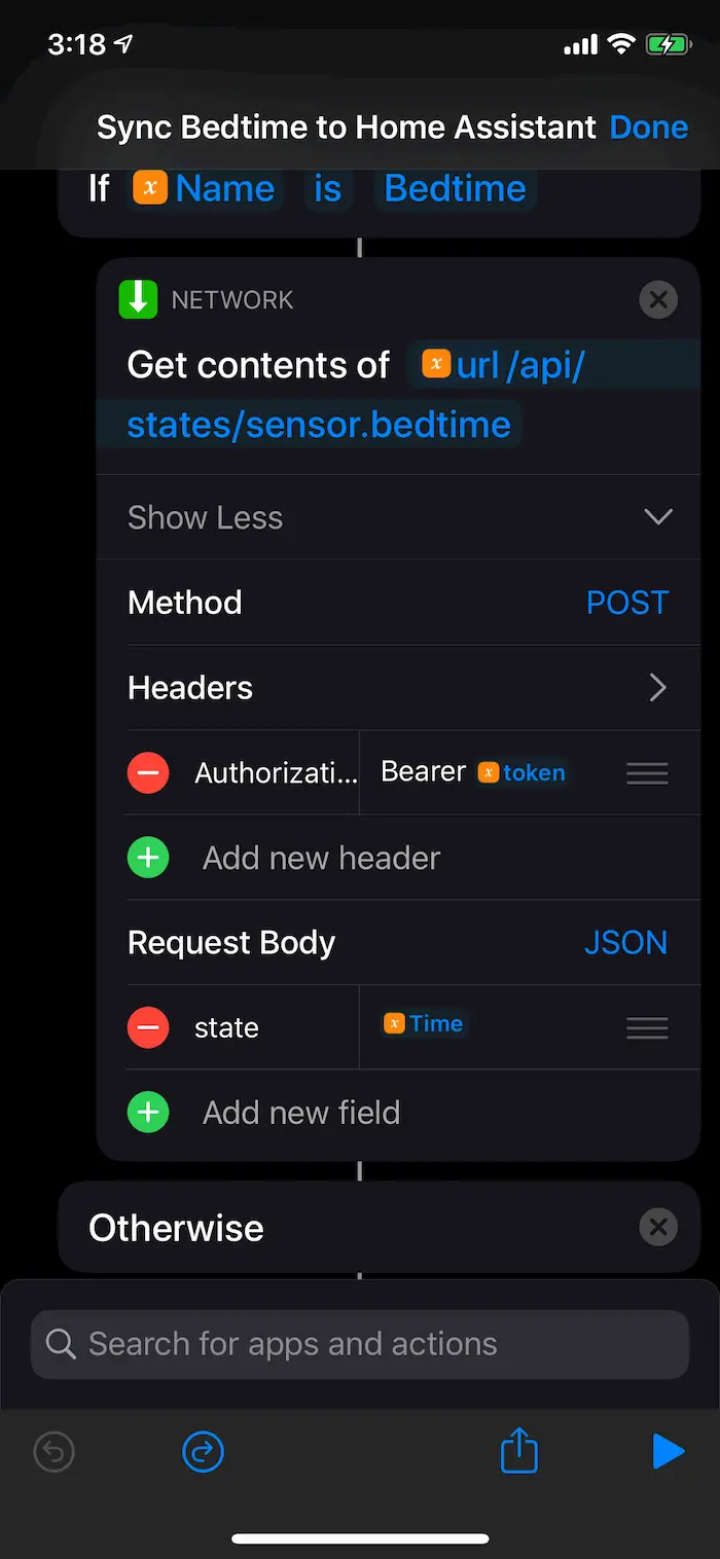The image depicts a cell phone screen with a black background, displaying various elements and text in white, blue, gray, red, green, and orange font. At the top, there are indicators showing 3 out of 18 bars for cell signal and Wi-Fi, and a battery icon that is fully charged in green. 

The main text reads: "Sync bedtime to home assistant done." Below this, it further elaborates with: "Name: bedtime. If name is bedtime, network: Get contents of URL API /states/sensor.bedtime. Show less method: post, headers." 

To the right, there is a red circle with a white line, indicating a missing or required authorization token. Below this is a green circle with a plus sign, prompting the user to "add new header." Further down, the text continues with: "Request body: JSON." This is followed by a red circle with a white line labeled "state," and another green circle with a plus sign to "add new field." Beside it is an "X" icon on the right side.

At the bottom of the screen, there's a search bar labeled "Search for apps and actions," accompanied by the standard cell phone navigation buttons for back, home, and recent apps, along with an icon of a box with an arrow pointing up and a right-facing triangle.

The overall color scheme includes shades of black, white, blue, gray, red, green, and orange, contributing to a visually complex interface focused on syncing bedtime data with a home assistant.